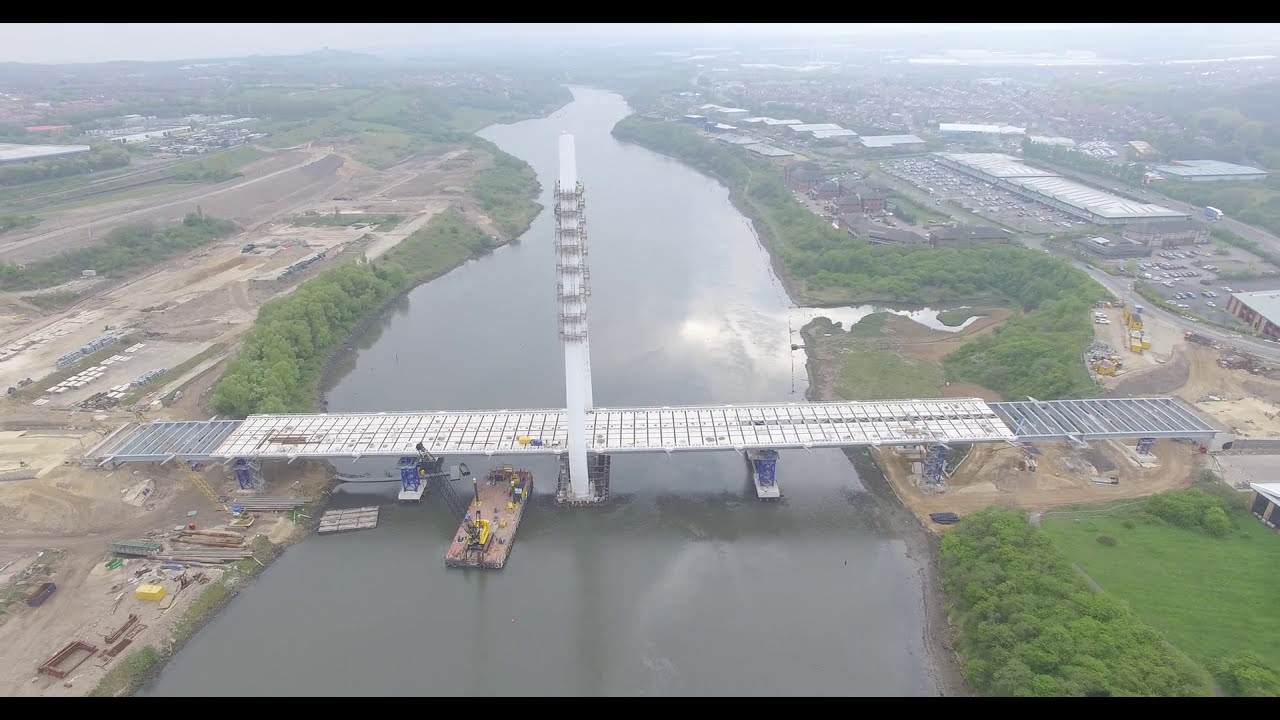The aerial image depicts the early stages of a bridge's construction spanning a river that flows from the bottom toward the top of the frame. The bridge, primarily composed of white metal parts, stretches across the river from left to right, with a substantial portion already in place, although the sides for the road are not yet constructed. Central to the bridge is a prominent tall pillar, likely for suspension cables. Below, light brown barges equipped with yellow construction machinery assist the work crew. The scene is dominated by expansive cleared areas of brown sand, with trees and greenery lining the riverbanks. Additional construction equipment is stationed on both sides of the river. In the background, buildings and parked cars can be seen, and the uppermost part of the image captures the sky. A grassy field lies to the bottom right, adding a natural element to the industrious landscape.